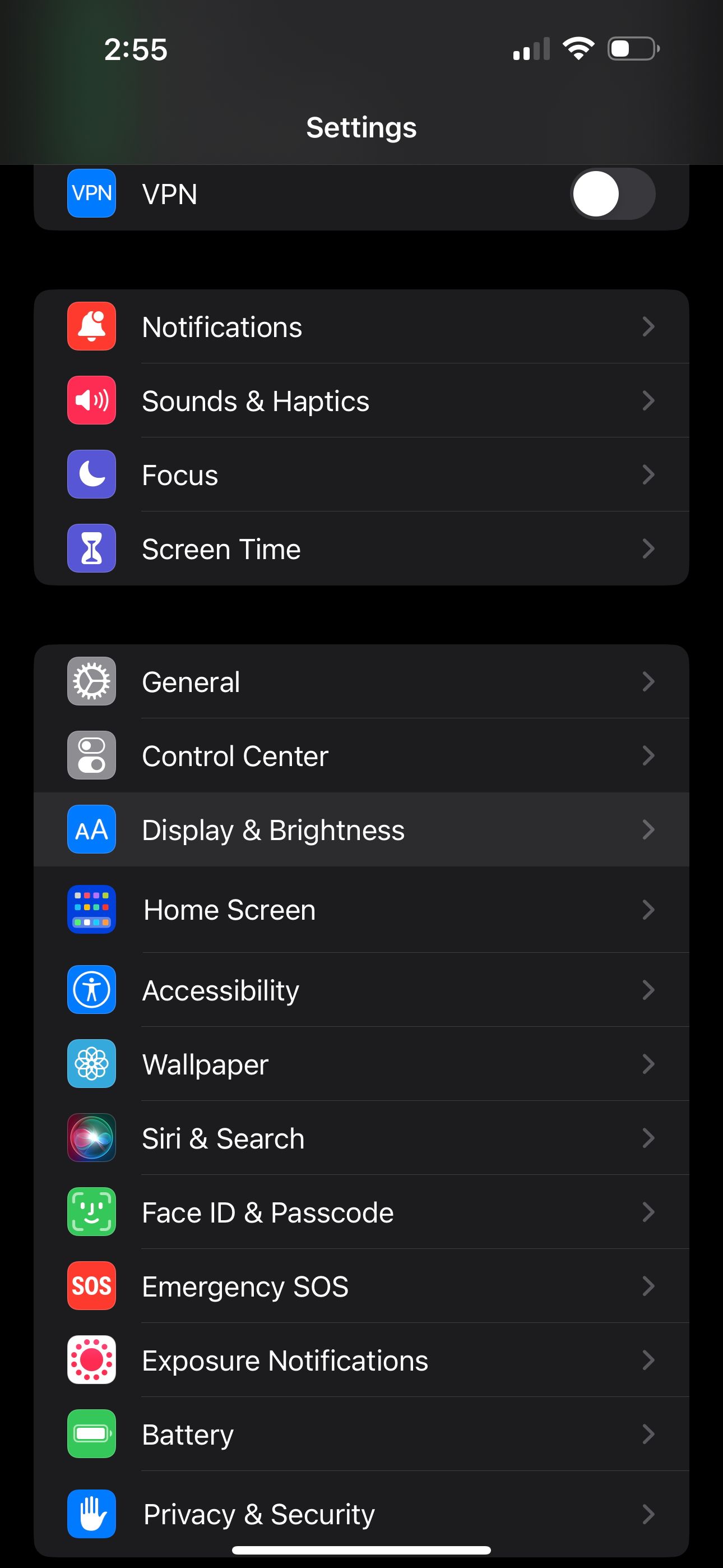A screenshot from a tablet or smartphone set to military time displays the time as 02:55 at the top. The right-hand corner includes status indicators: a cell signal at 2 out of 5 bars, a full Wi-Fi signal, and a battery indicator showing a little more than a quarter charged. The center of the screen prominently features "Settings" in white text.

The interface is sectioned into multiple settings categories:

1. **VPN Settings:**
   - A blue square with "VPN" in white text both inside and outside the square.
   - A grey, black mixture slider to the left, and a white circular toggle.

2. **Notifications:**
   - An orange background with a white bell and white circle.
   - "Notifications" written next to a gray arrow.

3. **Sounds & Haptics:**
   - A red square with a white speaker and curved white lines emanating from it.
   - "Sounds & Haptics" written next to a gray arrow.

4. **Focus:**
   - A purple square with a white moon.
   - "Focus" written next to a gray arrow.

5. **Screen Time:**
   - A purple square with an hourglass partially filled with purple sand.
   - "Screen Time" written next to a gray arrow.

The next major section contains additional settings options:

1. **General:**
   - A dark gray square with a white arrow inside.
   - "General" written beside it.

2. **Control Center:**
   - A gray square with sliders on the left and right.
   - "Control Center" written beside it.

3. **Display & Brightness:**
   - A dark blue square with two capital "A"s, one smaller than the other.
   - "Display & Brightness" selected.

4. **Home Screen:**
   - A dark blue square with multiple colored squares (white, red, purple, green, teal, cyan blue, orange, and mid-blue).
   - "Home Screen" written beside it.

5. **Accessibility:**
   - A dark blue square with a white circle containing a silhouette of a person.
   - "Accessibility" written beside it.

6. **Wallpaper:**
   - A cyan-blue square with a white atom symbol.
   - "Wallpaper" written beside it.

7. **Siri & Search:**
   - A black and red square with a circle divided into green, red, and blue segments.
   - "Siri & Search" written beside it.

8. **Face ID & Passcode:**
   - A green square with a white face symbol and little square bands emanating from it.
   - "Face ID & Passcode" written beside it.

9. **Emergency SOS:**
   - An orange square with "SOS" in white text.
   - "Emergency SOS" written beside it.

10. **Exposure Notifications:**
   - A white square with numerous smaller red dots around a larger central red dot.
   - "Exposure Notifications" written beside it.

11. **Battery:**
   - A green square with a white battery icon.
   - "Battery" written beside it.

12. **Privacy & Security:**
   - A dark blue square with a white hand icon.
   - "Privacy & Security" written beside it.

At the bottom, a white, oval-shaped, rounded rectangle navigation bar is visible, typical for iOS devices.

In summary, this screenshot provides a comprehensive view of various settings within an iPhone’s settings menu, showcasing a mix of security, privacy, and utility options, all detailed with distinct icons and background colors for easy identification.